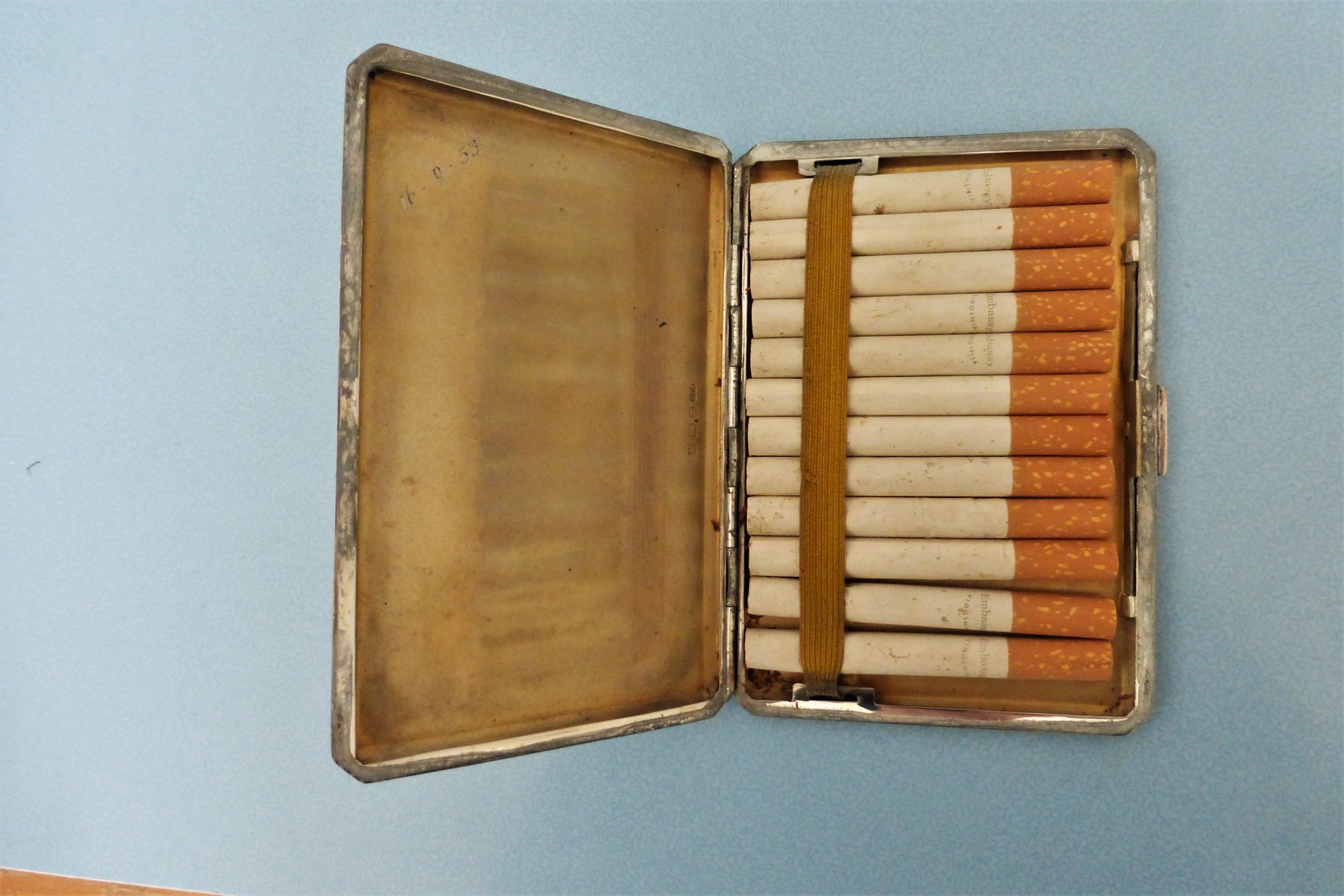This photograph showcases an old-fashioned silver metal cigarette tin, opened and resting on a smooth, light blue textured surface. The lid of the tin is hinged on the left side and is positioned open towards the left, with the bottom half containing the cigarettes on the right side. A clasp on the right side of the tin is visible, previously securing the lid. Inside, 12 cigarettes are neatly arranged horizontally, with their white bodies on the left towards the hinge and brown filters on the right near the clasp. These cigarettes are secured by a dark brown elastic strap situated closer to the white ends. The inner lid is also dark brown, providing a distinct contrast against the silver case and the light blue background. The metal case shows signs of age, with visible oxidation, adding to its antique appearance.